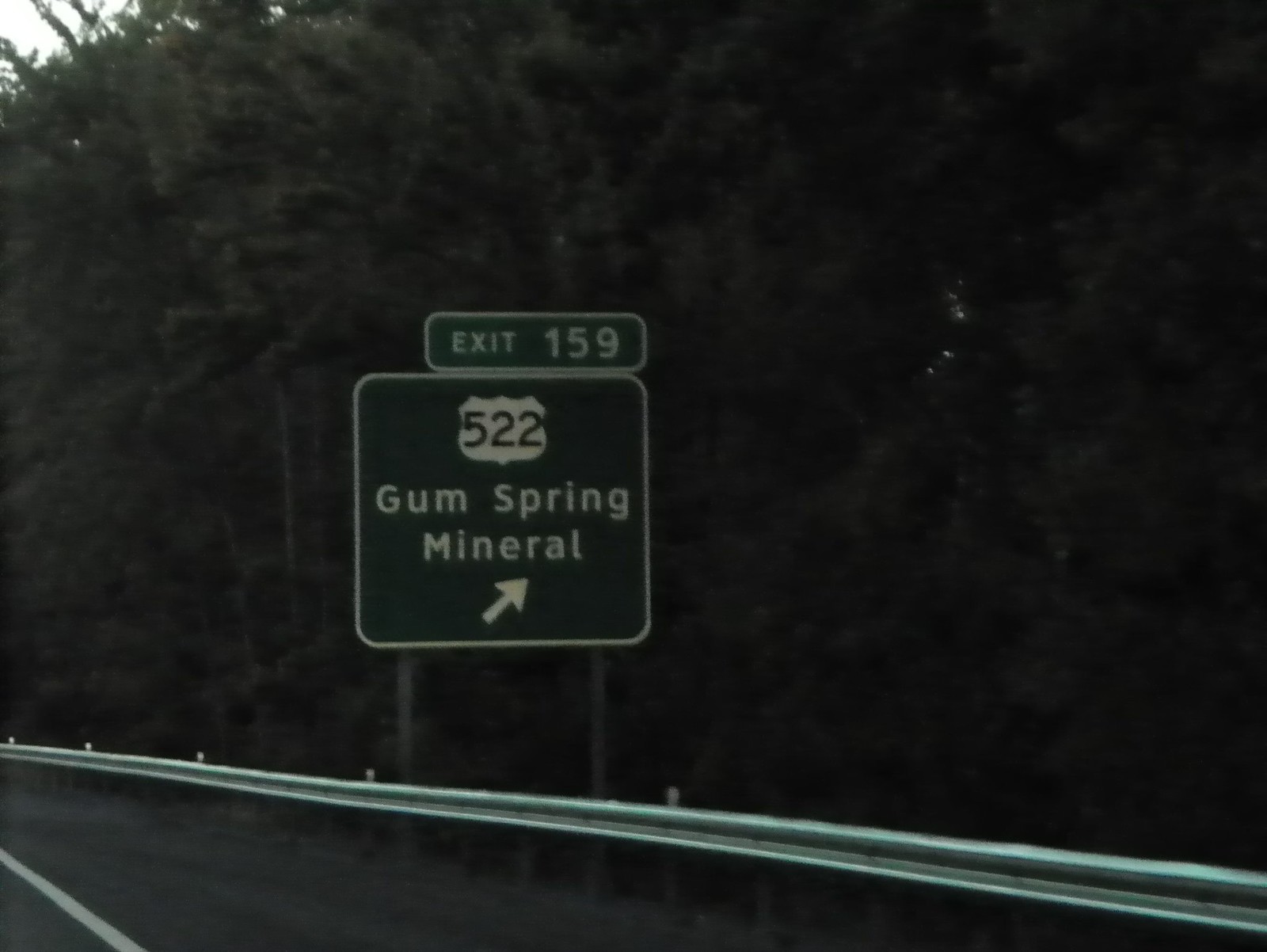The photograph appears to be taken from inside a car, revealing a scene dominated by a dense, wooded area with dark, almost silhouette-like trees. In the bottom left corner, there is a glimpse of the roadway marked by a white line, indicating a two-lane highway. Adjacent to this is an all-metal guardrail that separates the road from the forest. The focal point is a large street sign located just behind the guardrail. The sign is composed of two main parts: a rectangular sign on top that reads "Exit 159," and a larger square sign below it that indicates "Highway 522" with an arrow pointing up and to the right, suggesting a northeast direction. Beneath this, the sign also reads "Gum Spring Mineral." The image, though dark and somewhat gloomy, features a tiny patch of light-colored sky peeking through the dense foliage, adding to the moody ambiance of the scene.